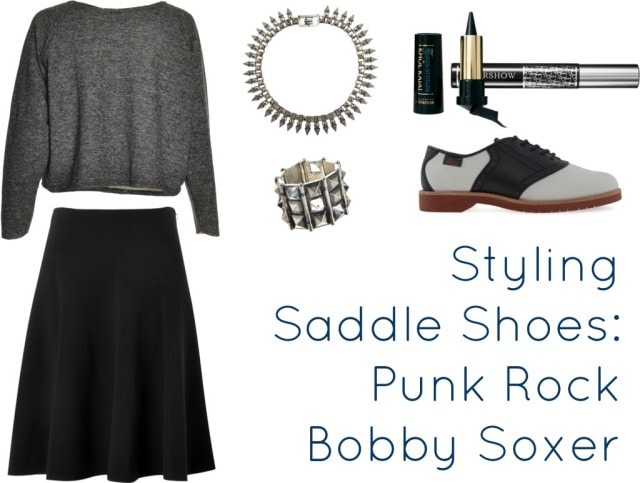The image features a collection of apparel and accessories arranged in a square pattern against a white background. In the upper left corner is a charcoal gray long-sleeve sweater. Below the sweater is a solid black long skirt. To the right of these garments, there is a silver metal bracelet and a metal ring. In the upper right corner, you'll find a silver tube of mascara lying on its side and a tube of black lipstick with a triangular point, housed in a gold and black base. Below these items, near the bottom right, lies a black-and-white saddle shoe with a brown sole, facing right. Some black text is situated in the lower right side of the image, reading "styling saddle shoes: punk rock Bobby Soxer." This text seems to label the collection of items displayed.